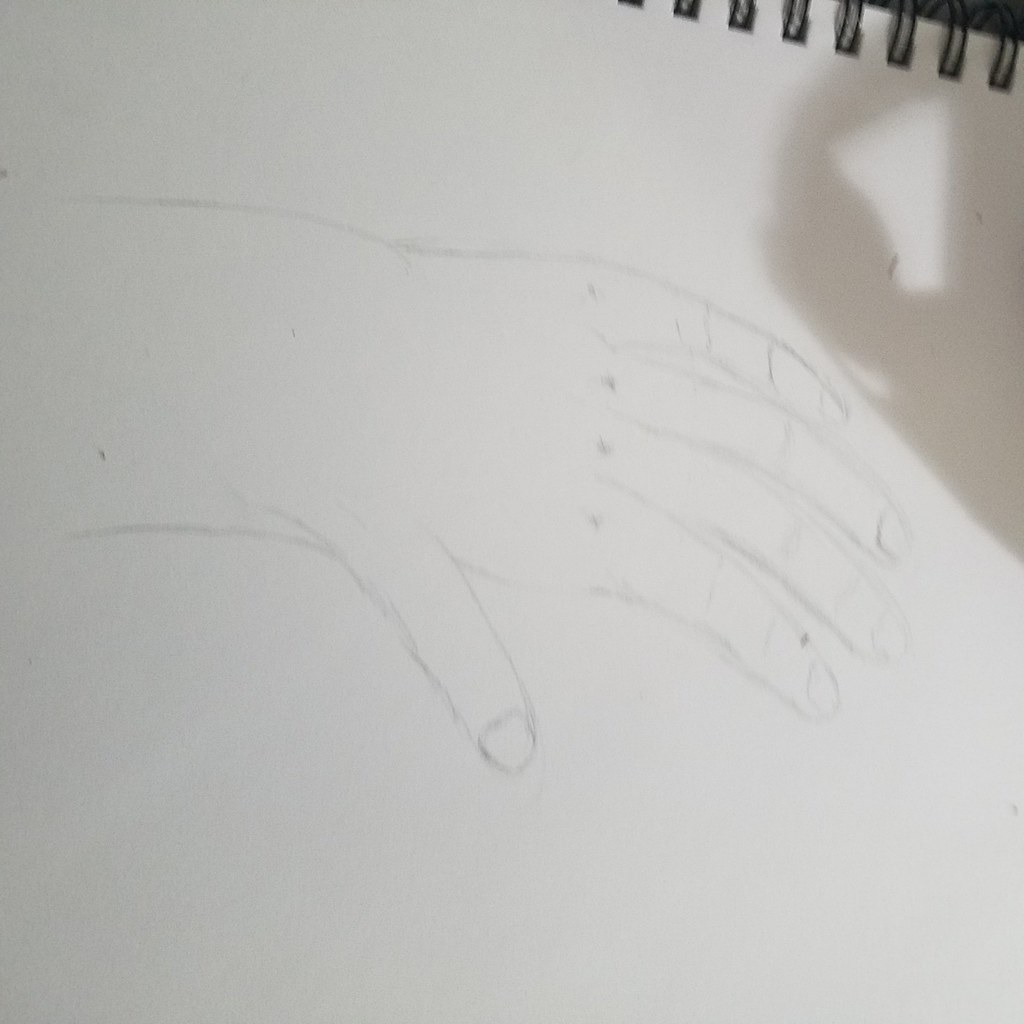A detailed drawing of a left hand is depicted on a sketch pad with black, wired binding, which appears at the top right of the image due to the slanted perspective. The hand, illustrated with four fingers and a thumb, extends from the upper left side of the composition. The wrist and a small portion of the forearm are also visible. Each finger is marked with a dot to indicate the knuckles, adding a touch of anatomical detail to the artwork.